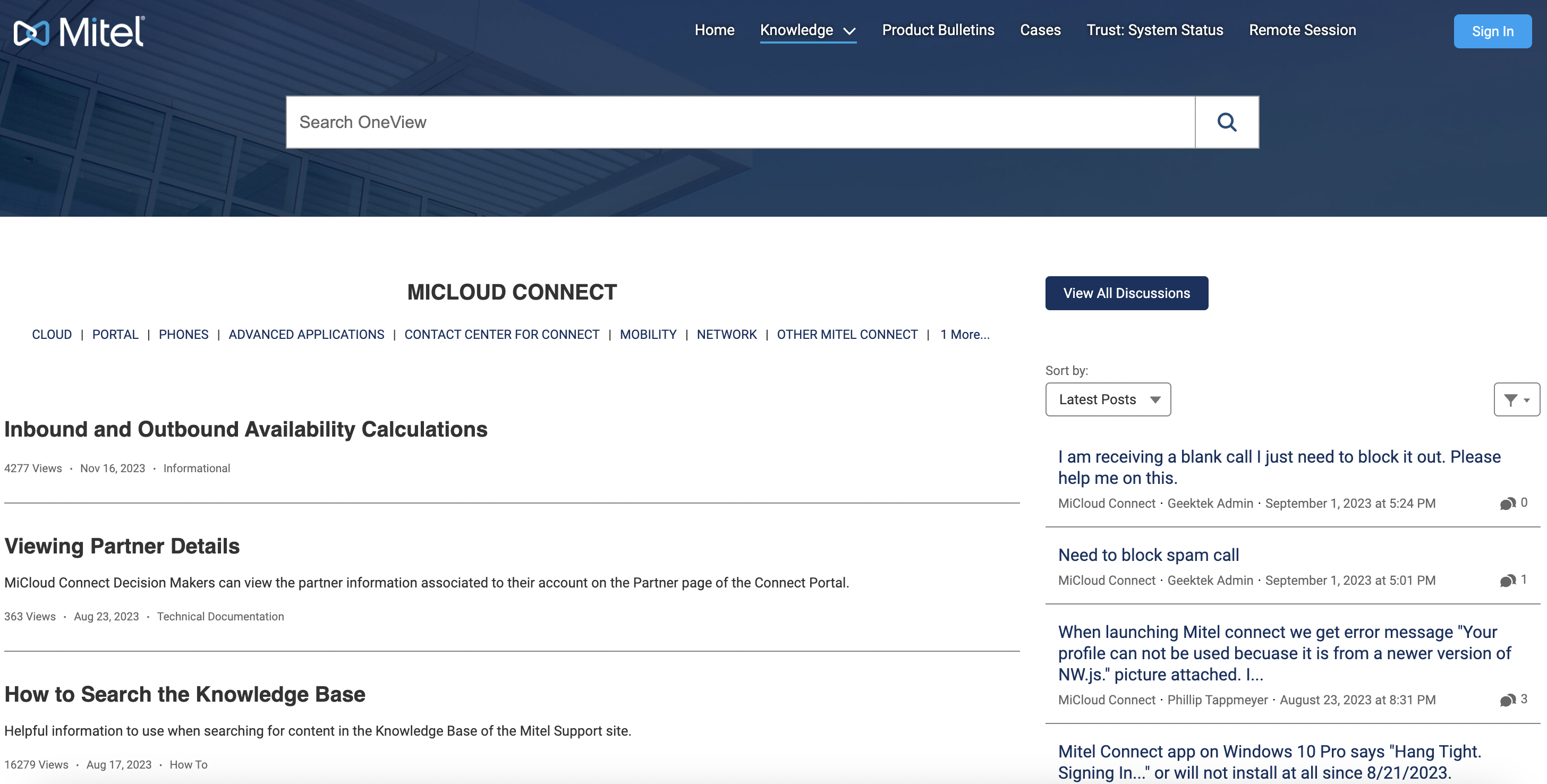In the image, the top left corner features the word "METEL" written in white, next to an icon of two interlocked triangles, with the left triangle being white and the right one blue. The right side of the image displays a navigation menu with tabs titled HOME, KNOWLEDGE, PRODUCTS, BULLETINS, CASES, TRUST, SYSTEM STATUS, REMOTE SAVING, and a blue SIGN IN button at the top right corner. Below the button is a search box labeled "SEARCH ONE VIEW" set against a slightly dark blue background. 

The left side of the page shows a section titled "MY CLOUD CONNECT." Under this heading, there are several tabs in blue: CLOUD PORTAL, PHONES, ADVANCED APPLICATION, CONTACT CENTER FOR CONNECTS, MOBILITY NETWORK, ADAMETER CONNECT, among others. Beneath these tabs, there is black text that reads "UNBOUND AND ADBOUND AVAILABILITY CALCULATION FOR THE 277 VIEWS NOVEMBER 16, 2023 INFORMATIONAL."

Additional text details are provided, including: 
- "VIEWING PARTNER DETAILS, MY CLOUD CONNECT DECISION MAKERS CAN VIEW THE PARTNER'S INFORMATION ASSOCIATED TO THEIR ACCOUNT ON THE PARTNER PAGE OF THE CONNECTS PORTAL, 363 VIEWS AUGUST 23, 2023 TECHNICAL DOCUMENTATION"
- "HOW TO SEARCH THE KNOWLEDGE BASE, A HELPFUL INFORMATION TO USE WHEN SEARCHING FOR CONNECTED KNOWLEDGE BASE OF THE METEOR SUPPORT SITE, 16,279 VIEWS AUGUST 17, 2023 HOW TO."

On the right side, there is a "VIEW ALL DISCUSSIONS" section displaying four discussion topics:
1. "I'M RECEIVING A BLANK CALL, IF I JUST NEED TO BLOCK IT OUT, PLEASE HEAD ME ON THIS. THERE IS NEED TO BLOCK SPAM CALL."
2. "WHEN LAUNCHING METEOR CONNECT, WE GET AN ERROR YOUR PROFILE CANNOT BE USED VERSION OF NW.JS."
3. "METEOR CONNECT APP ON WINDOWS 10 PRO SAYS HANG TIGHT, SIGN IN OR WILL NOT INSTALL AT ALL SINCE 8, 21, 2023."